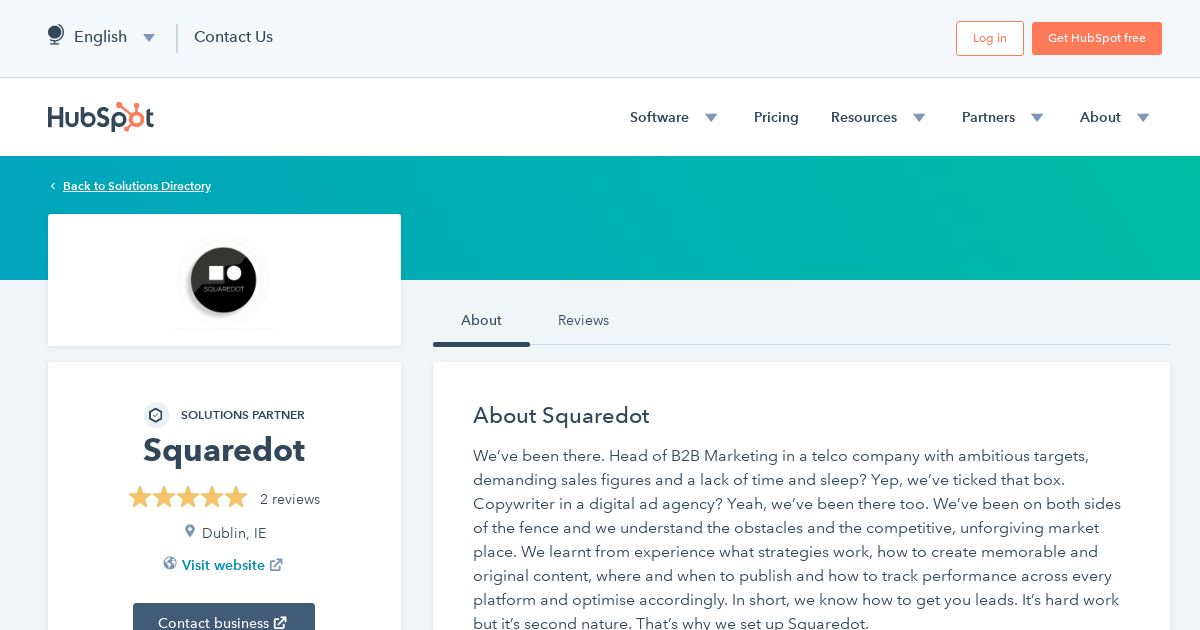The screenshot from the HubSpot site offers a detailed view of its navigation and content. At the top of the page, several tabs are available for users, including:

- **Software** (accompanied by a drop-down arrow)
- **Pricing**
- **Resources** (accompanied by a drop-down arrow)
- **Partners** (accompanied by a drop-down arrow)
- **About** (accompanied by a drop-down arrow)

At the bottom, a blue banner stretches across the screen, featuring a "Back to Solutions Directory" option on the left side. 

Scrolling down, the highlighted **About** page is underlined, with a **Review** section adjacent to it. The content on the **About** page reads:

> **About Square Dot**
> 
> We've been there: head of B2B marketing in a telco company with ambitious targets, demanding sales figures, and a lack of time and sleep. Yep, we've ticked that box. Copywriter in a digital ad agency? Yes, we've been there too. We've worked on both sides of the fence and understand the obstacles in the competitive, unforgiving marketplace. Our experience has taught us which strategies work. We know how to create memorable and original content, determine the best times and platforms for publishing, track performance, and optimize accordingly. In short, we know how to generate leads. It's hard work, but it’s second nature to us. That's why we established Square Dot.